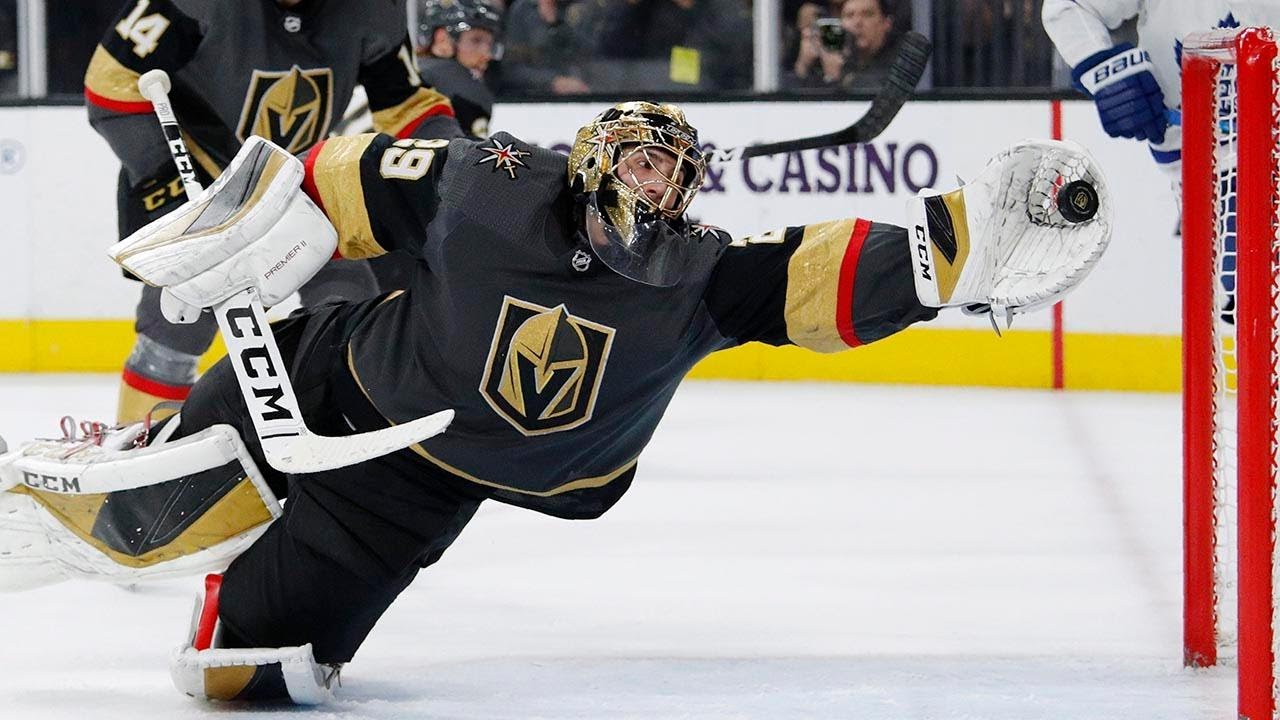A dynamic moment captured in mid-action shows a hockey goalie dramatically reaching out to catch a puck in his white glove, just before it sails into the red goal situated on the right side of the image. The goalie appears to be leaping backward, exhibiting remarkable agility. He is donned in a full goalie uniform, featuring a distinctive golden black face mask helmet. His jersey is predominantly black, gold, and red, and prominently displays a helmet emblem with a gold "V" on the front. The goalie wields a large white goalie stick and is equipped with protective goalie pads. The ice beneath him glistens, capturing the intensity and speed of this frozen moment. In the background, partially obscured, is one of his teammates, shown from the chest up, along with the rival opponent wearing a white and blue uniform, showcasing only his glove. The backdrop includes the spectators in the stands, divided from the rink by a protective wall, adding to the atmosphere of a high-stakes hockey game.